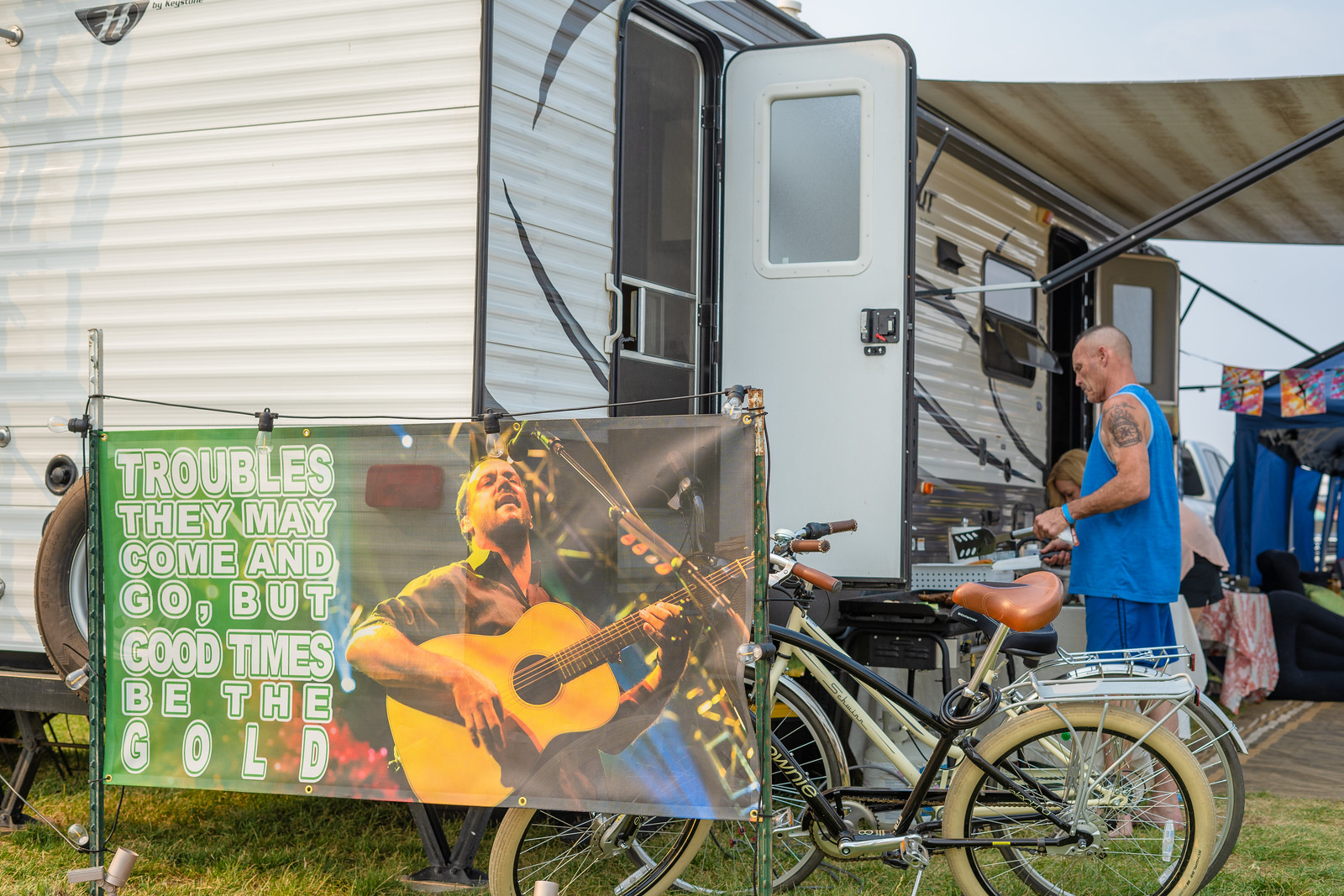The photograph captures a lively camping scene in a grassy area, centering around a white trailer, possibly a Winnebago or an RV camper, which has two open doors and an awning extending over one side. The trailer is adorned with lights, suggesting a festive atmosphere. Prominently displayed outside the trailer, on a canvas sign supported by two poles, is the phrase, "Troubles, they may come and go, but good times be the gold," written in green letters. Below the text is an image of a man playing a golden guitar, reminiscent of Dave Matthews from the Dave Matthews Band.

In front of the trailer, multiple activities are taking place. A man with dark blue shorts, a blue shirt, and a tattoo on his left arm is seen standing by a table cluttered with miscellaneous items, possibly grilling or barbecuing. Nearby, a tricycle with a brown seat and tan wheels and a pair of bicycles hint at recreational opportunities. To the side of the trailer, two more people are visible, including a woman standing behind the man, adding to the social setting. Laundry hangs on a line near the rear, and additional tents can be seen in the background, enhancing the sense of a communal camping event. The overall scene gives an impression of relaxed camaraderie and enjoyment.